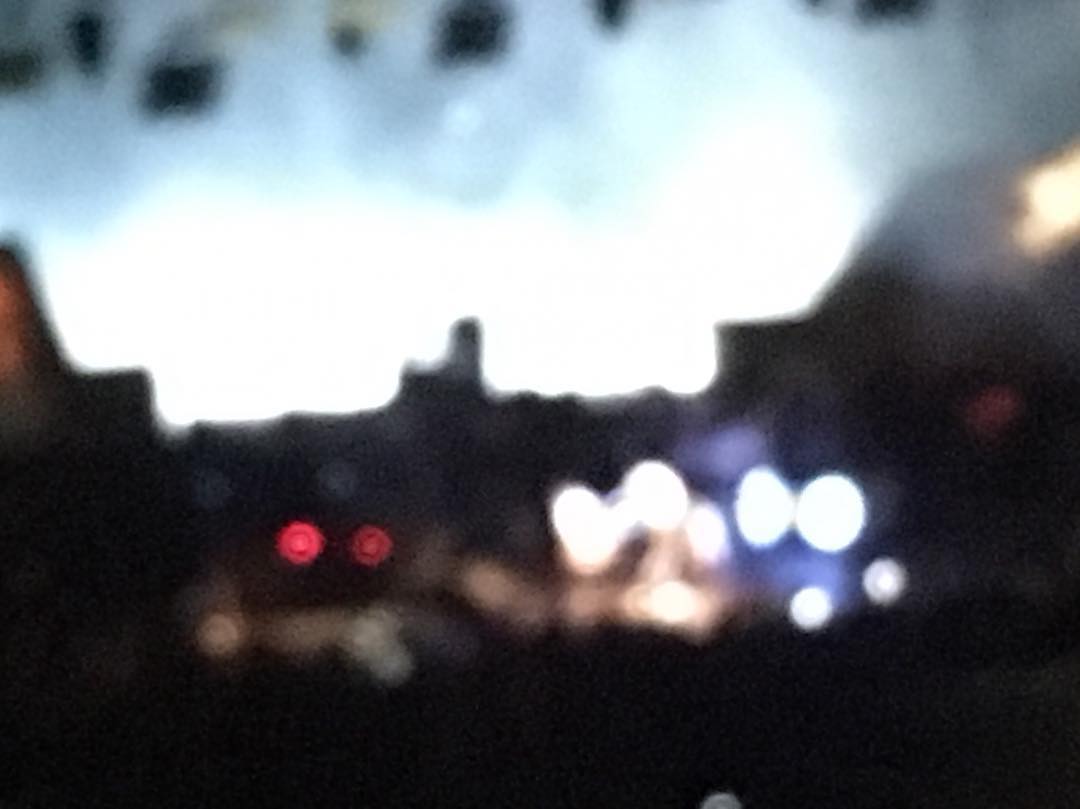The image appears to be taken at dusk, capturing the transitional moments from day to night. Although the image is blurry, one can make out an opening in the sky straight ahead, which showcases a blend of blue and white hues, possibly hints of the remaining daylight. The atmosphere in the forefront of the image is relatively dark, with various lights punctuating the scene. Notably, there are two distinct red lights, side by side, resembling glowing eyes, which create an intriguing focus. To the right side of the image, bright white lights can be seen in the distance, adding another layer of interest. The viewpoint suggests that this photograph might have been taken from inside a vehicle, contributing to the blurriness and the scattered light effects.